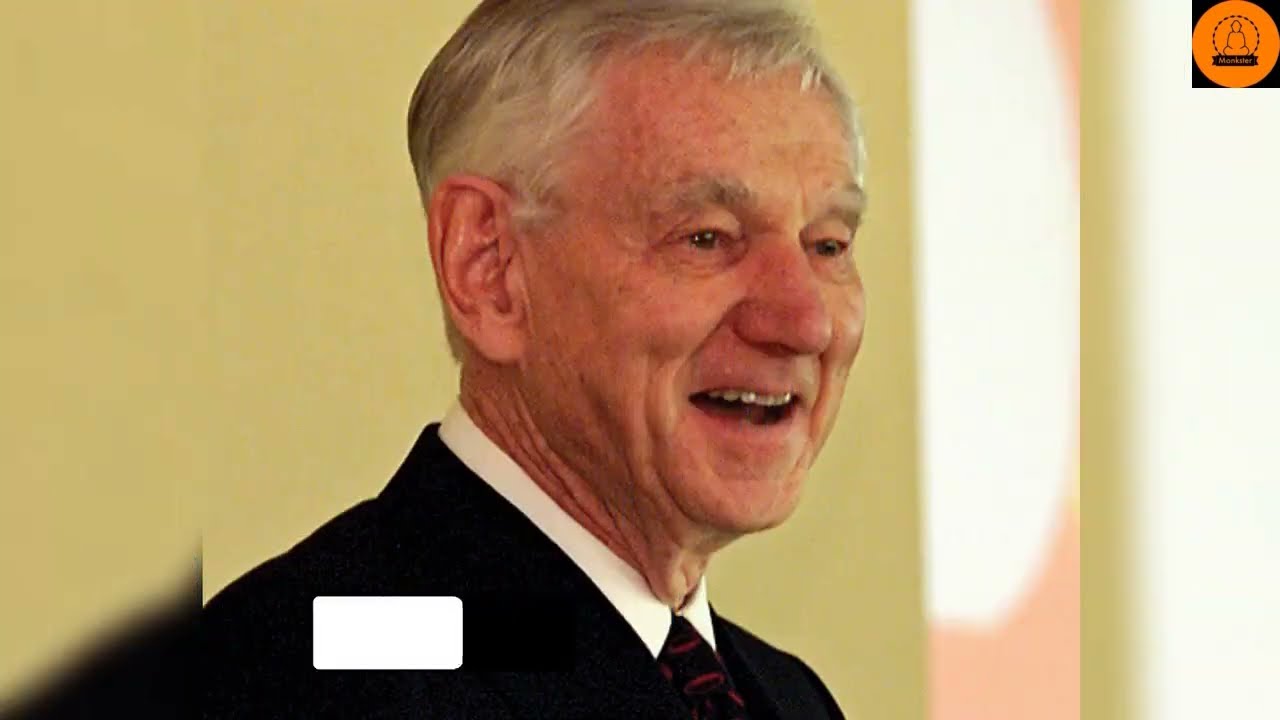This photo captures an elderly gentleman named David Murdoch, who appears to be in his 70s or approaching his 80s. The image is a head-and-shoulder portrait featuring David in a black suit, complemented by a white shirt and a black tie with red stripes. His short gray hair, interspersed with bits of white, mirrors the color of his eyebrows. He has prominent ears and a warm smile revealing his top teeth, as he looks slightly to the right. In the background, there is a yellow wall with a soft light shining from the right, and a distinctive white, rounded square behind him. Additionally, in the top right corner of the image, a black square with an orange circle and the word "Monkster" can be seen, adding a unique element to the backdrop.